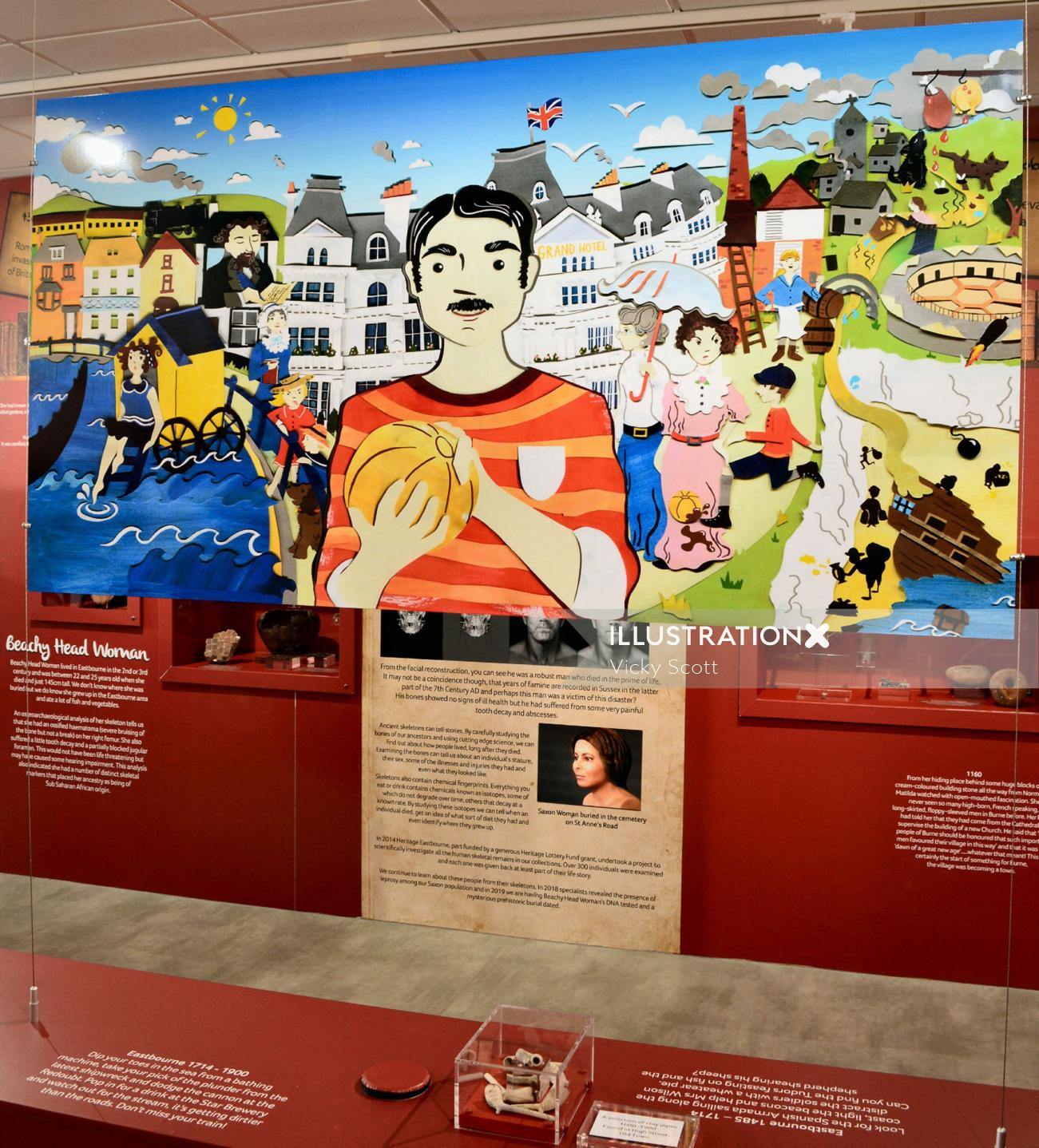This vibrant and detailed mural, created by Vicki Scott and titled "Beachy Head Woman," is prominently displayed in a museum environment. The artwork, characterized by its bright colors and vintage 1920s aesthetic, showcases a central figure—a man with a mustache and short black hair, wearing a red and orange striped shirt with a white shield logo on the breast pocket. He holds a beach ball. Notably, a UK flag tops a large white building in the background, reminiscent of a Grand Hotel. To the left, a woman dips her toe into a bay of water, adding to the whimsical scene. Various other figures with umbrellas can be seen throughout, adding life to the joyful cityscape. This mural is suspended over a red exhibit explanation panel, complete with white text detailing various exhibits, and is surrounded by other artifacts in the museum. A yellow sun can be seen in the top left corner, illuminating the vibrant colors of the painting.